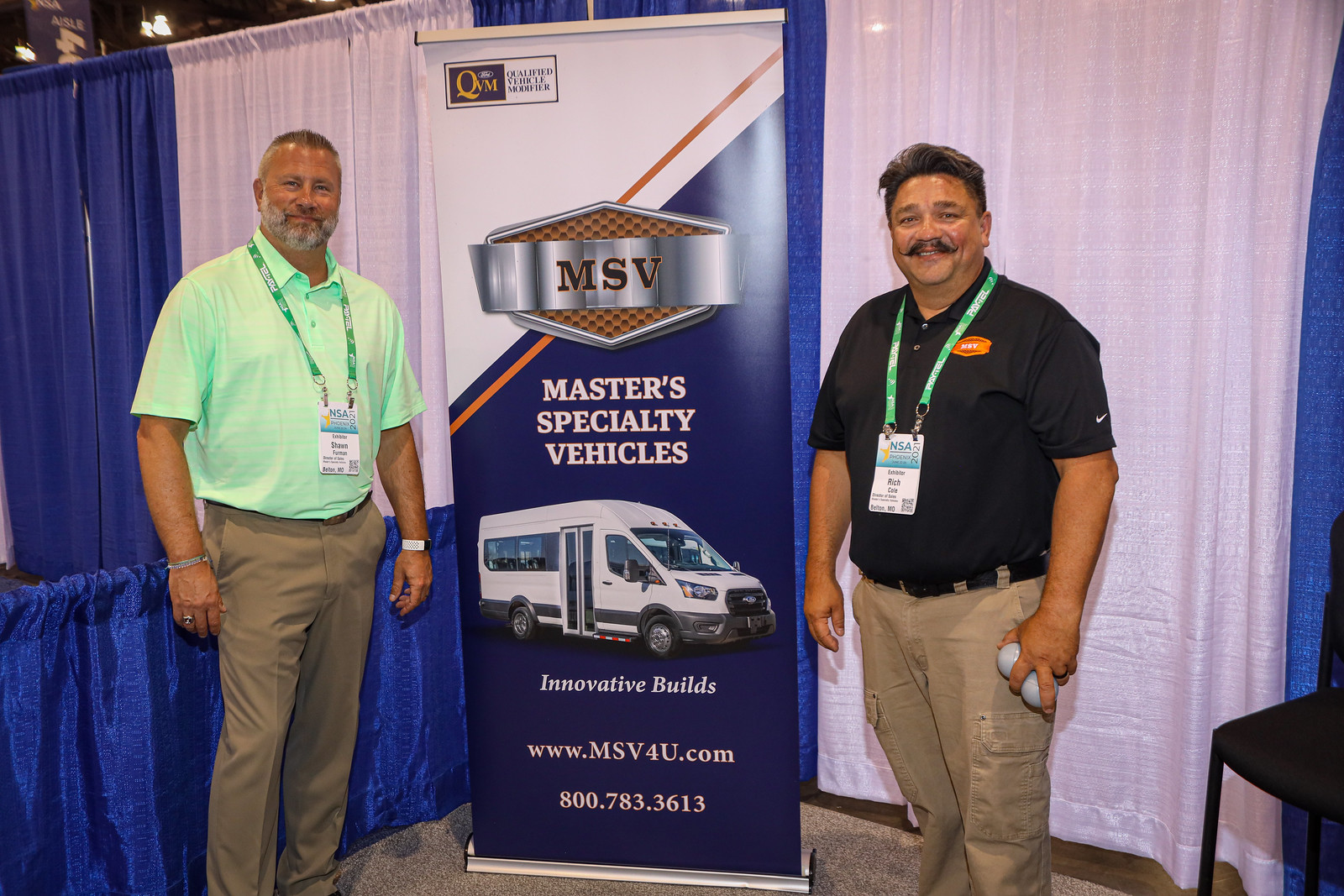This color photograph, likely taken at a convention or trade show, features two men standing on either side of a large poster advertisement for MSV Masters Specialty Vehicles. The backdrop is a series of alternating blue and white curtains. The man on the left is tall and is dressed in a lime green short-sleeved polo shirt paired with khaki dress slacks. Notably, he accessorizes with a bracelet and a ring on his right hand, a white-banded wristwatch on his left hand, and a green and white lanyard with an identification card around his neck. He has very short brown hair, a gray beard, and a friendly smile, indicating he is likely Caucasian. The man on the right, shorter in stature, is wearing a black short-sleeved Nike polo shirt, identifiable by the emblem on his left arm, also paired with khaki slacks and a black belt. He sports short black hair, a black mustache, and wears a similar green and white lanyard with an ID card. He appears to be Latino. The central advertisement showcases a small bus or recreational vehicle and reads, "MSV Masters Specialty Vehicles Innovative Builds," with the website www.msv4u.com and the phone number 800.783.3613 clearly visible at the bottom. Both men are smiling broadly, suggesting they are enjoying the event.